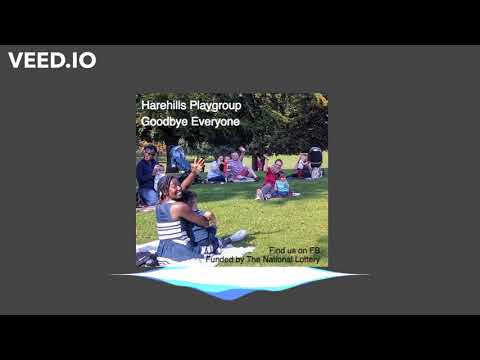This color photograph captures a lively picnic scene of parents and children seated on green grass, enjoying their time together. Everyone is sitting on picnic blankets, with parents either holding their children or having them by their sides. In the foreground, a woman in a blue and white dress is waving to the camera, a young child on her lap. Behind them, more people, including a woman in a red shirt with a child and a man in a long sleeve black and blue shirt with gray pants, are also facing the camera. The backdrop includes a few trees, contributing to the park setting.

Embedded over the image is text: the top left corner of the photograph reads "Hare Hills Playgroup, Goodbye everyone" in white font, while the bottom right says, "find us on FB, funded by the National Lottery." The entire photograph is set against a solid dark gray background, with additional white text in the top left corner spelling "VEED.IO." There are also black bands at the top and bottom of the picture, adding a framed effect. Beneath the image, a small decorative white graphic further embellishes the scene.